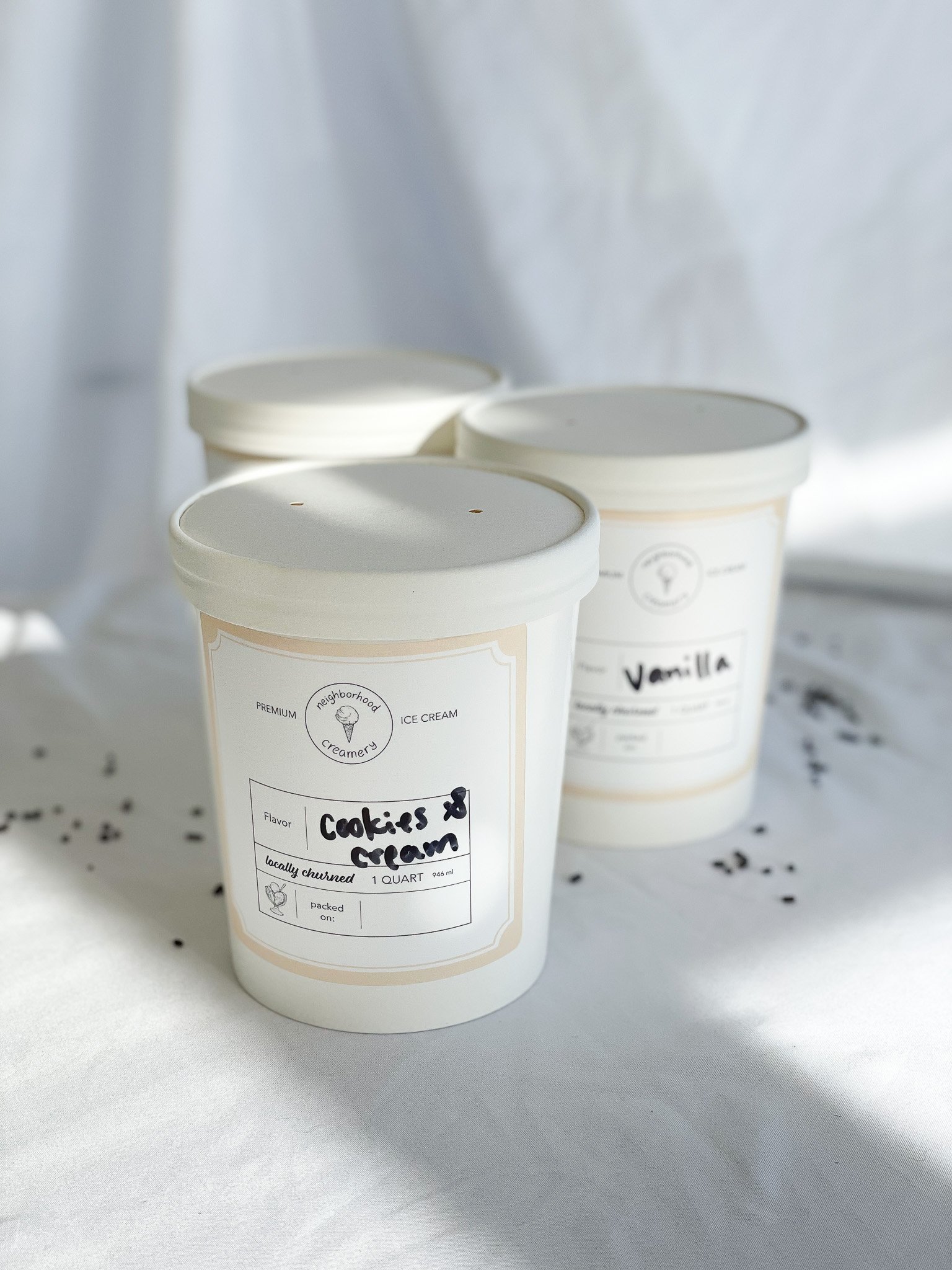This detailed color photograph depicts three cartons of ice cream, neatly arranged against a white, somewhat pleated, and wrinkled cloth backdrop. The ice cream containers, each one quart in size, sit on a table draped with the same white cloth. The prominent carton in the foreground proudly displays its label, which reads "Premium Neighborhood Creamery Ice Cream," followed by the handwritten flavor "Cookies and Cream." Further details include "Locally Churned, One Quart, 946 ml," and a drawing of a dish of ice cream with an incomplete "Packed on" date. Just behind the foreground carton, a second carton, slightly blurred, is labeled "Vanilla." The third carton in the back is mostly obscured by the first two. Scattered around the cartons are numerous small brown and black specks, resembling crumbs or sprinkles, adding a touch of texture to the otherwise pristine setting.